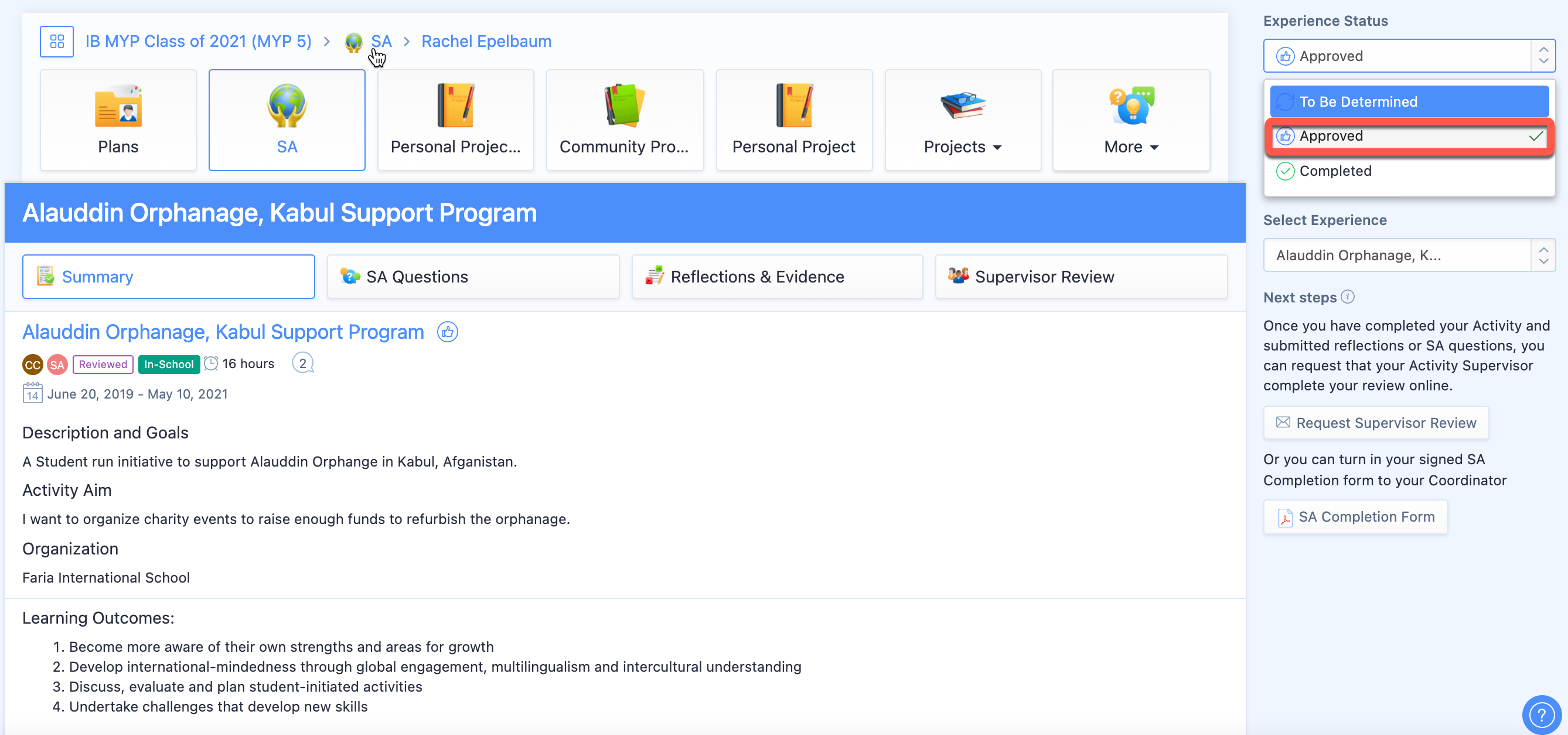Here is a clean and detailed caption for the described image:

---

The web page displays the IB MYP Class of 2021 (MYP5). At the top, icons and text are aligned with arrows pointing to the right, featuring a depiction of hands holding up a globe and the letters "SA." Following this, the name "Rachel Eppelbaum" is prominently displayed. 

Beneath this header, six to seven rectangular buttons are labeled "Plans," each accompanied by various icons. The headings under these icons include "SA," "Personal Project," "Community Pro," "Personal Project," "Projects and More." 

Further down, a blue banner with white text reads "Lawdon Orphanage, Kabul Support Program." Below this banner, a series of white rectangles contain headings for different sections: "Summary," "Essay Questions," "Reflections and Evidence," and "Supervisor Review."

Another blue banner below repeats the title "Lawdon Orphanage, Kabul Support Program," followed by a detailed paragraph outlining the description, goals, activity aim, organization, and learning outcomes of the project. 

To the right of this descriptive paragraph, a sidebar menu displays the "Experience Status" as approved within a white rectangle. It continues with the text "To be determined," followed by the word "Approved" circled in red. 

Further options in this menu allow for selecting experiences, with a white rectangle labeled "Lawdon Orphanage K." Below, it mentions "Next Steps" with an accompanying paragraph detailing the forthcoming actions. At the bottom right corner of the page, a help icon is shown as a white question mark inside a blue circle.